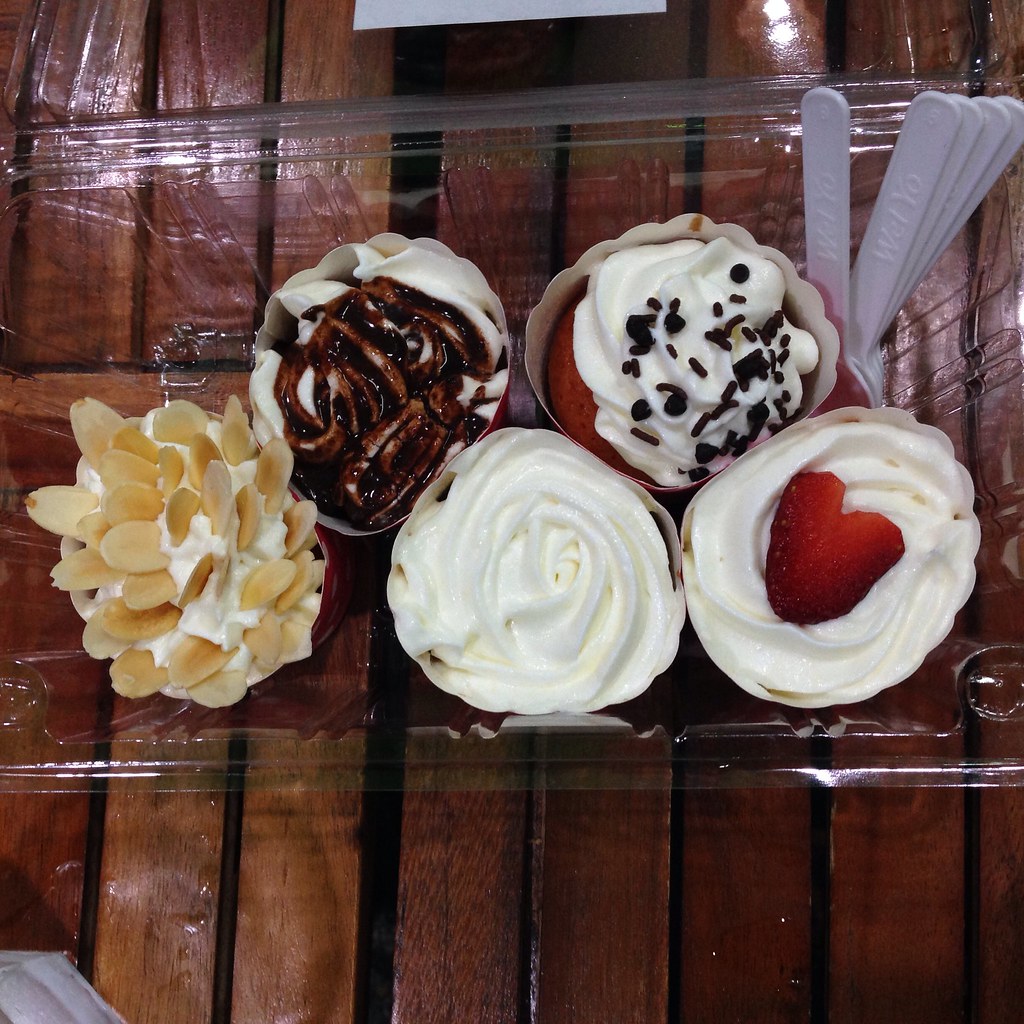This realistic photograph captures a clear plastic tray placed on a picnic table made of dark brown wooden planks arranged vertically. In the tray, there are five cupcakes, organized with two on the top row and three on the bottom row, viewed from above. In the top right corner of the tray lie the handles of five white plastic spoons, although the spoon parts are not visible. The cupcakes exhibit a variety of decorations: the bottom left cupcake is topped with white whipped cream and almond slivers, the bottom center one has plain white whipped cream, and the bottom right shows white whipped cream adorned with a strawberry. On the top row, the cupcake to the left features white whipped cream with black sprinkles, possibly over red velvet cake, and the top right cupcake has white whipped cream drizzled with chocolate sauce. The spoons have illegible white text printed on them.